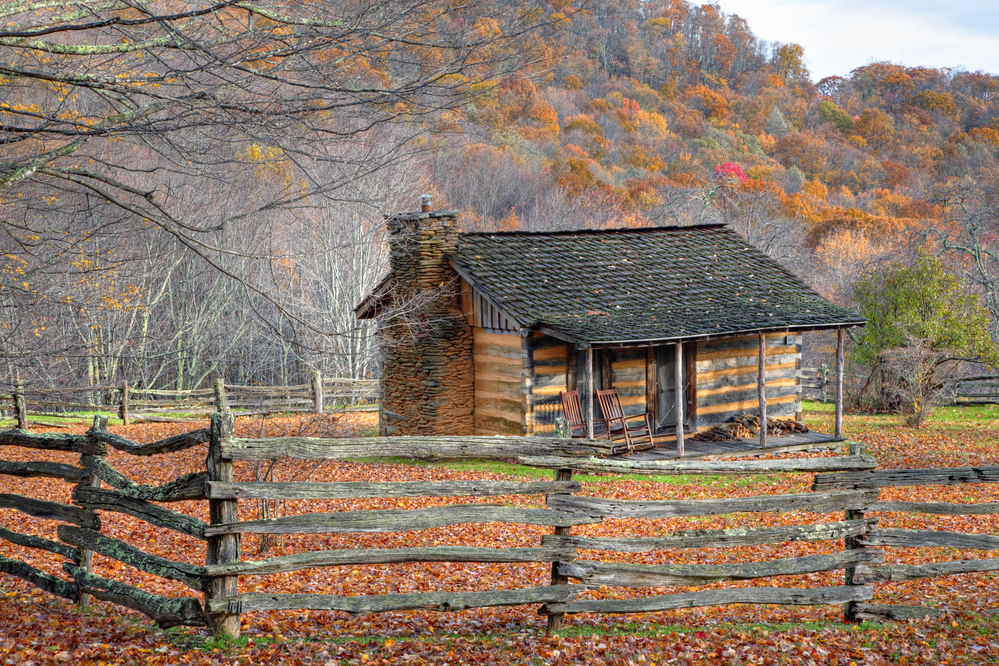The image depicts a highly detailed painting of a small, rustic shack or cabin situated in a serene rural area, surrounded by the vivid colors of autumn. The cabin, constructed from brown wooden logs with a distinct black roof and a chimney on its left side, is central to the scene. It is slightly angled towards the right, providing a view of the inviting front porch, which features two wooden rocking chairs. 

In the foreground, the cabin is enclosed by a wooden fence that appears to be crafted from raw, unrefined logs, giving it a natural, rugged charm. This fence is constructed with five horizontal beams and vertical poles spaced roughly ten feet apart, standing around four feet high.

The ground within the fenced area is littered with red and orange leaves, indicative of late fall. Surrounding the fenced yard, the background is densely populated with trees displaying a stunning array of fall foliage, ranging from orange to dark red. A particular tree in the upper left corner stands bare, adding to the seasonal atmosphere of the painting. This picturesque scene captures the tranquility and beauty of a rural autumn landscape.